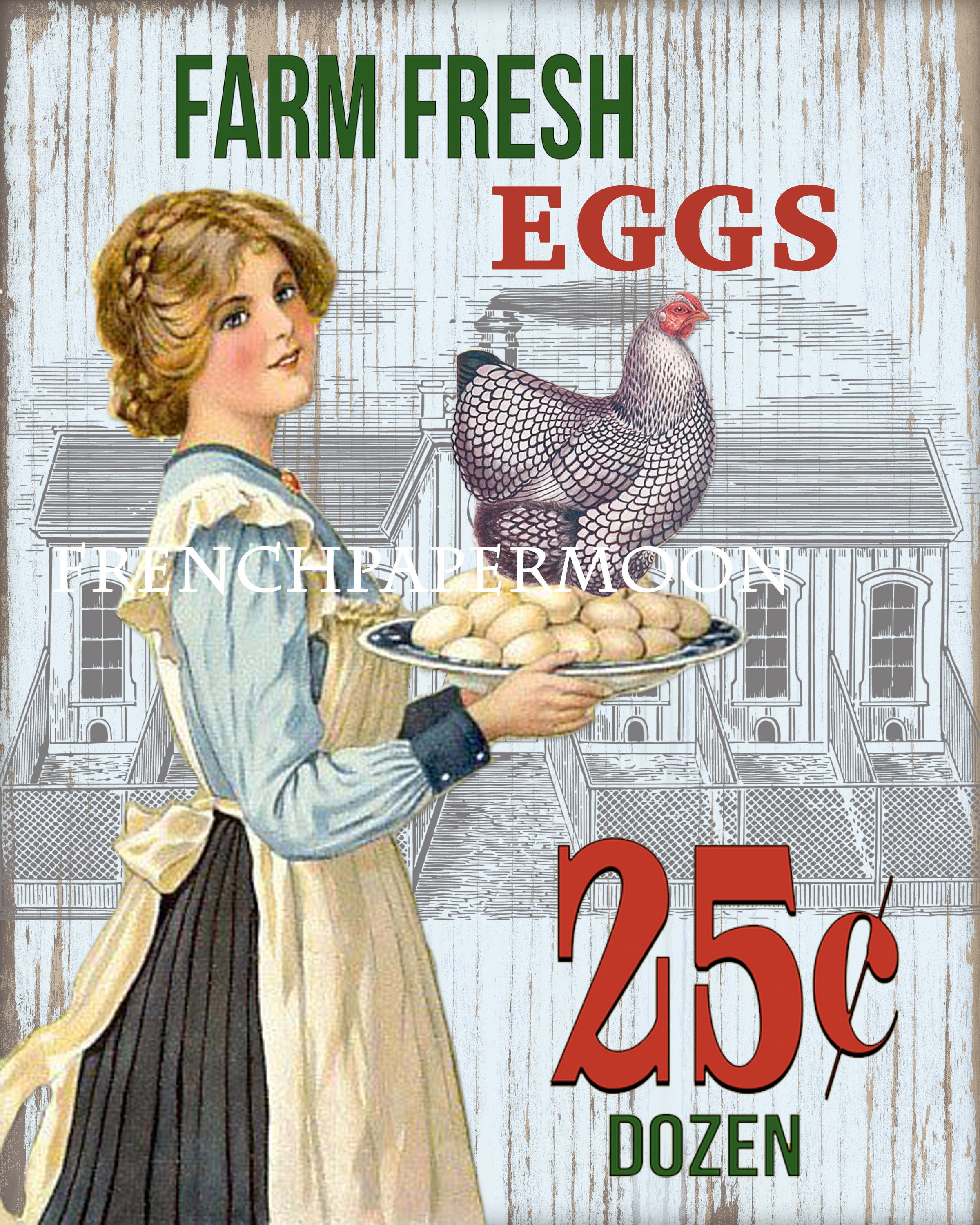The advertisement showcases a young woman with red hair tied in a braid, dressed in a colonial-style outfit consisting of a long tan apron with ruffled sleeves, a blue long-sleeve shirt, and a long black skirt. She is holding a large platter filled with eggs, on which a hen with a grid-like pattern stands. The text "Farm Fresh Eggs" is prominently displayed at the top, with "Farm Fresh" in green and "Eggs" in red. At the bottom right, it states "25 cents a dozen," with "25 cents" in red and "a dozen" in green. The background features a worn, wooden texture and a black-and-white illustration of a barn, complete with chicken coops, wire runs, and small holes for the chickens to access the outdoor enclosures. The woman is positioned facing right while looking at the viewer, adding an old-fashioned, rustic charm to the scene.